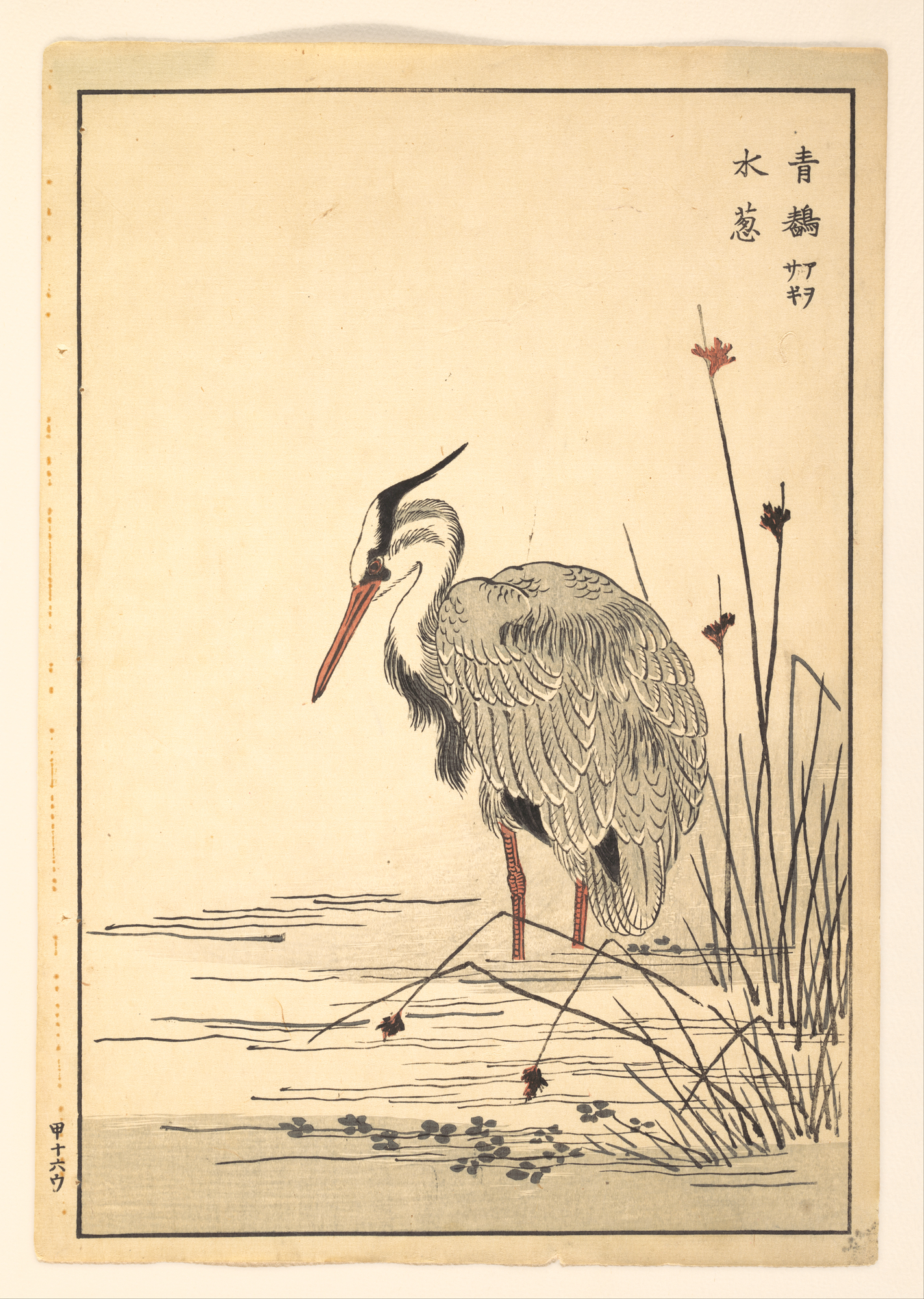This is a detailed sketch on off-white, slightly beige, rectangular paper, oriented vertically. The artwork depicts a large bird, likely a crane or heron, standing in water. The bird's body is primarily shaded in gray, with large gray feathers adorning its back and wings. It has a distinct white neck and head, accented with subtle light gray shading. Both the bird's beak and legs are vividly colored in orange, contrasting with the monochromatic body. The legs are partially submerged, blending into the water, which is stylized with simple black ripples. To the right of the bird, a few delicate blades of grass or plants emerge from the water, accompanied by a couple of clover-like leaves. The style of the drawing is reminiscent of traditional East Asian art, perhaps Chinese or Japanese, with black ink used predominantly. In the upper right-hand corner, there is text written in what appears to be a foreign script, possibly Chinese or Japanese characters, adding an authentic cultural touch to the piece.